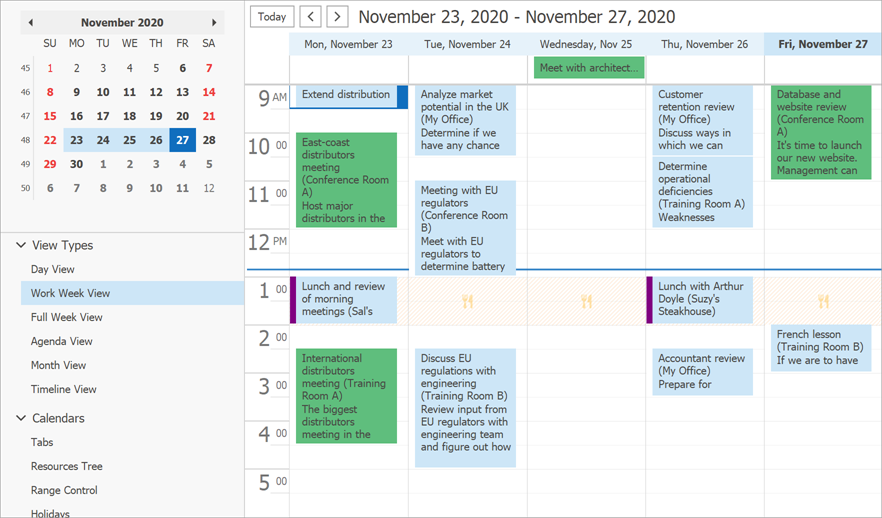The image shows a calendar in the top left corner marked with "November 2020," where the date "27th" is specifically highlighted. The calendar interface includes various view options listed as "Day View," "Work Week View," "Full Week View," "Agenda View," "Month View," and "Timeline View." The calendar appears in a blue-highlighted "Full Week View" mode. Additional features such as "Calendar Tabs," "Resource Tree," and "Range Tree Control" are also visible, alongside a panel for "Holidays."

The main section of the calendar covers the week from November 23, 2020, to November 27, 2020, detailing each day from Monday the 23rd to Friday the 27th. The time slots range from 9 a.m. to 5 p.m. 

On Friday, the 27th, the schedule is bold and includes multiple tasks such as:
- "Extend Distribution"
- "Meet Architect"
- "Customer Retention Review"
- "Analysis Market"
- "East Coast Distributor Meeting"
- "Lunch and Review of Morning Meeting"
- "International Distributor Meeting"
- "Discuss EU Regulations with Engineering"
- "Accountant Review"
- "Lunch with Arthur Doyle"
- "French Lesson"
- "Determine Operational Deficiencies"
- "Weaknesses Determine Batteries"